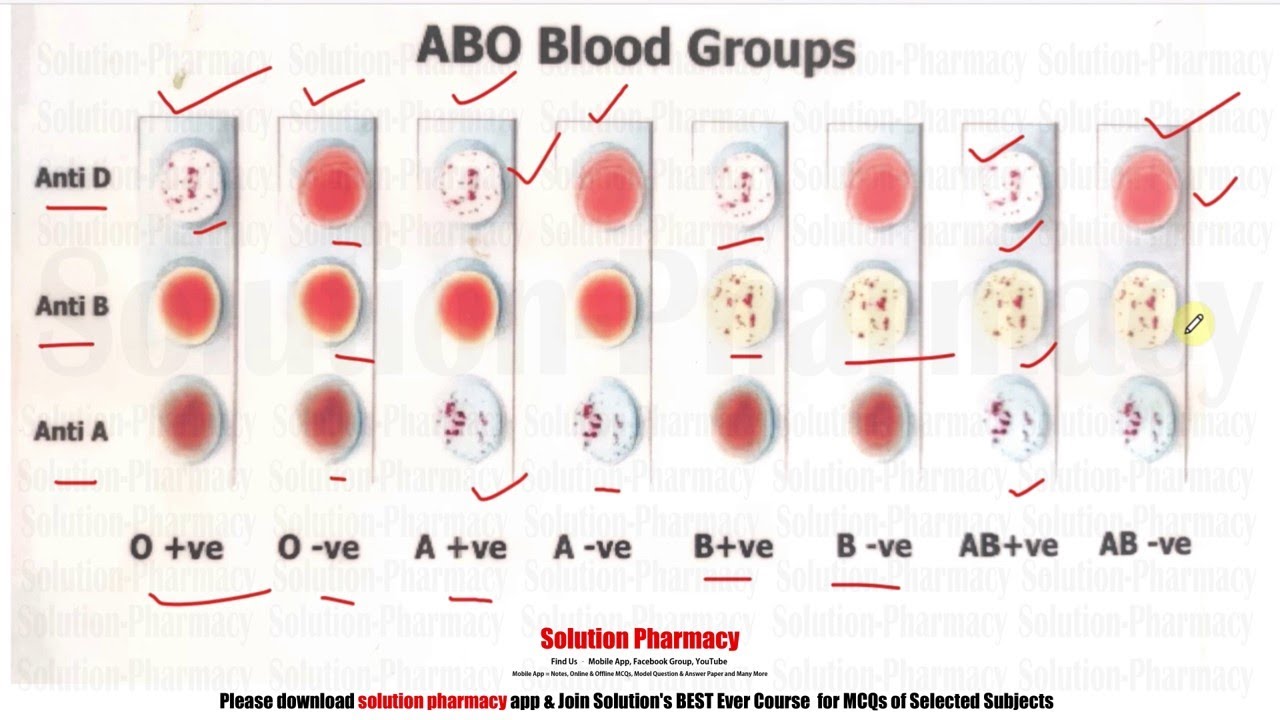The image is a horizontal, rectangular chart on a white background with the title "ABO Blood Groups" at the top in prominent black letters. The chart consists of rows labeled "anti-D," "anti-B," and "anti-A," and columns labeled with various blood types: O positive (O+), O negative (O-), A positive (A+), A negative (A-), B positive (B+), B negative (B-), AB positive (AB+), and AB negative (AB-). Different colored circles, red and yellow with red dots, are present in the chart indicating reactions or results associated with each blood type. Additionally, pencil and pen marks, including red check marks and black lines, are visible, suggesting that someone has used the chart for an explanation or annotation. At the bottom, in small red text, it says "Solution Pharmacy," accompanied by an invitation to download the Solution Pharmacy app and join their MCQs course for selected subjects.